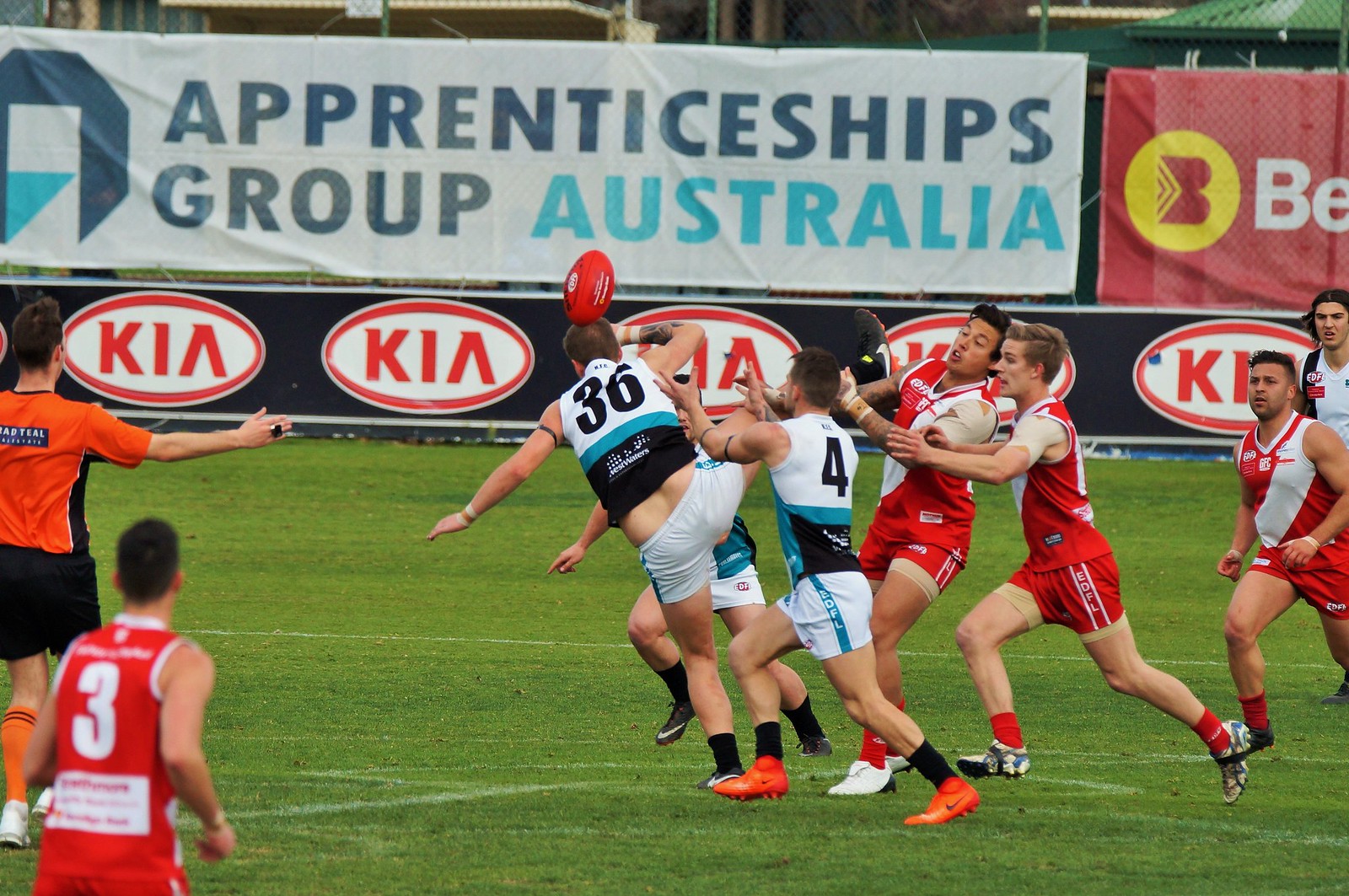This is an outdoor Australian rules football match, evident from the sleeveless jerseys and the distinct ball. The image captures a dynamic moment on the field where two teams, the teal, black, and white-clad players and their red and white opponents, converge at the center. The team sporting white tops with black and teal accents, and teal-striped white shorts stand poised as the red team, characterized by their predominantly red uniforms with distinctive white diagonal stripes, rush towards them. The football has just hit a player positioned in the center of the action, adding to the scene's intensity. Key advertisements, including a prominent Kia logo and a banner for Apprenticeships Group Australia, frame the background, adding commercial context to the lively scene. Additionally, an official in a red shirt with black shorts, marked by black stripes, is visible on the field, ensuring the game’s regulation. The match is set against a clear daytime sky, emphasizing the outdoor setting of this competitive and spirited Australian sporting event.